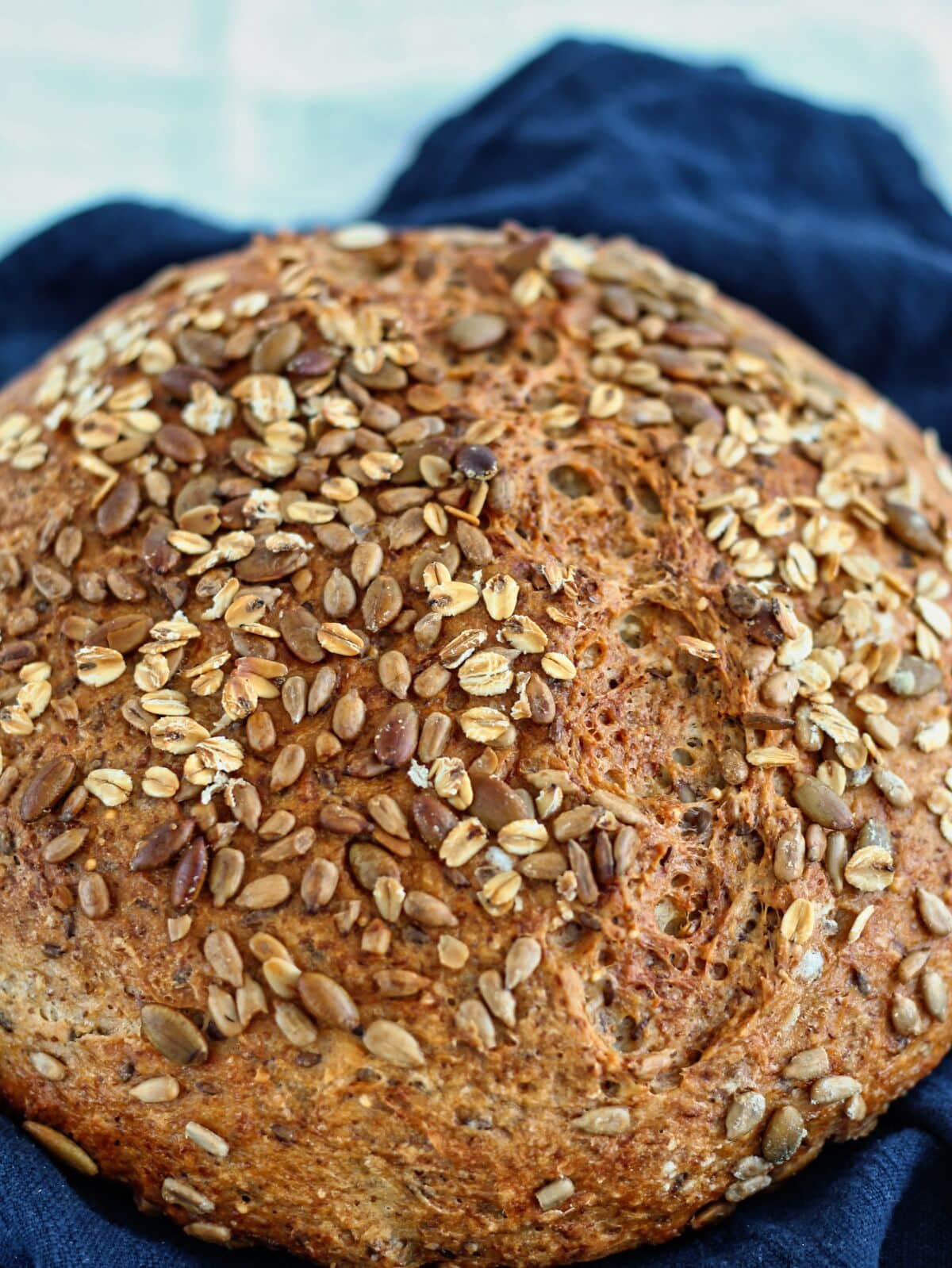The image is a close-up photograph of a round, dome-shaped whole grain bread roll with a dark brown crust. The bread roll is encrusted with an assortment of seeds, predominantly small pieces of oats, sunflower seed kernels, and other seeds ranging in color from light beige to dark brown. The seeds are more densely clustered on the top of the roll and become sparser towards the sides. A noticeable furrow, where the bread split open during baking, runs vertically along the right side. The bread roll stretches across the entire width of the image and occupies roughly three-quarters of its height. It rests on a dark blue towel, which is visible around the bottom left, bottom right, and top edges of the image. In the background, the light blue color of the setting provides a soft contrast. Shadows in the blue towel, particularly at the top and bottom right, suggest the presence of a light source illuminating the scene.